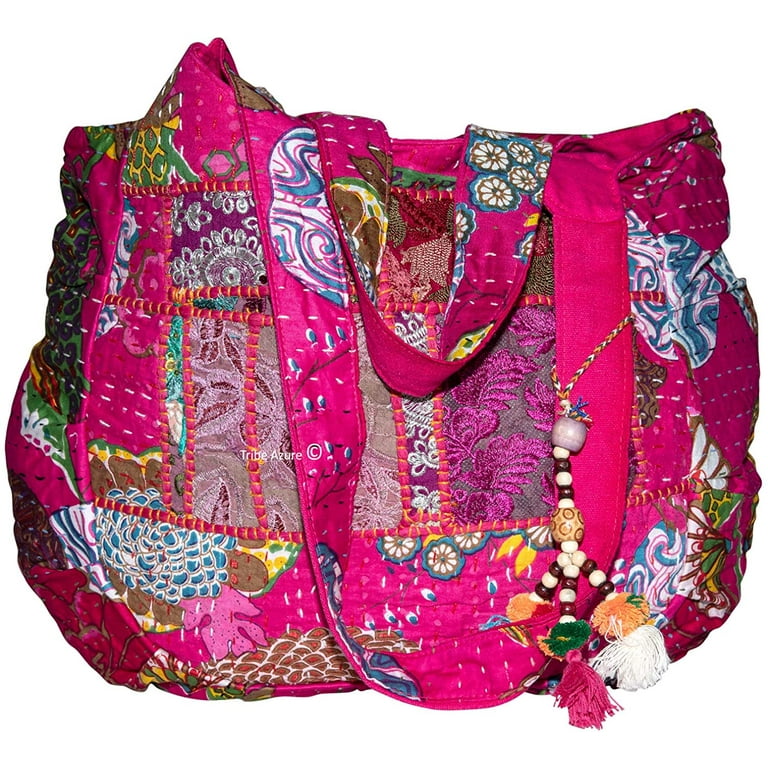This image showcases a handmade, oversized boho handbag crafted from a patchwork quilt. The bag is predominantly hot pink or magenta, with an array of vibrant sections featuring floral and circular patterns in colors such as blue, brown, purple, green, yellow, turquoise, and white. The handbag sports two thick shoulder straps, with a distinctive beaded decoration hanging from one of the straps. This bead decoration includes brown, gold, and white beads, interspersed with colorful tassels in shades of pink, white, orange, and green. The fabric has a slight shine, adding to its textured and multi-colored appearance. Detailed stitchwork in white and yellow is evident throughout the bag. Additionally, in the center of the image, the brand name "Tribe Azure" is visible, confirming the artisan quality of the piece, all set against a solid white background.